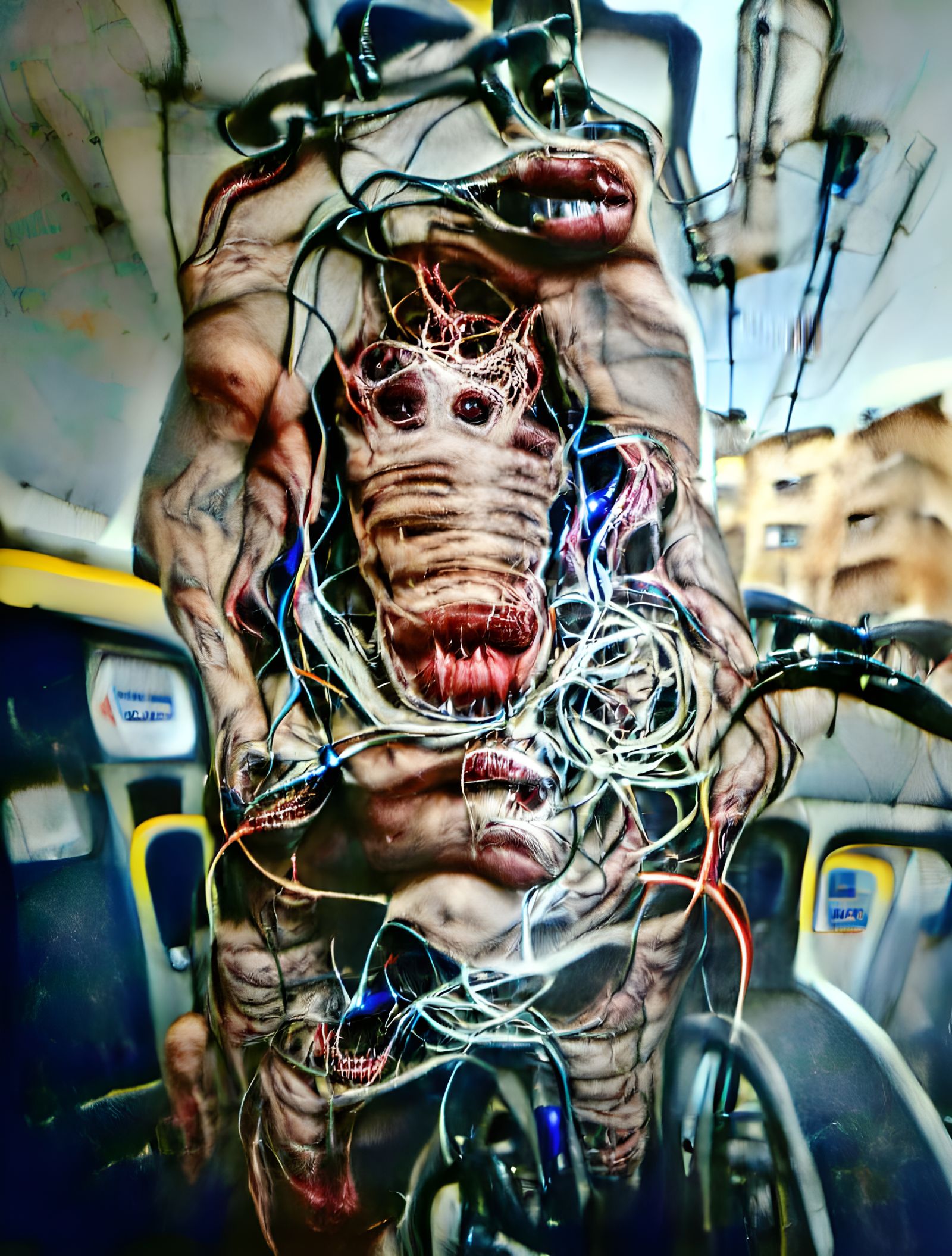The image is an abstract, likely AI-generated composition that defies conventional structures and presents a surreal, disturbing figure. Dominating the center is a flesh-toned entity intertwined with a chaotic mass of wires and veins. The upper portion, resembling limbs, ambiguously morphs into arms or legs, adding to the otherworldly sensation. Central to the composition are four or five eye-like cavities, positioned where a torso might be, with tumultuous ripples descending toward an uncanny, misplaced mouth below. Scattered across the body, which lacks clothing, are veins or wires in white, blue, and yellow hues, enhancing the sense of a biomechanical fusion. Another mouth is disturbingly situated around the area corresponding to the abdomen. The background, though blurred, hints at an exterior setting possibly like a townscape or bank, but it remains distorted and detached from reality. This disjointed amalgamation of body parts and wiring creates a monstrous, unsettling figure that challenges perception and makes an indelible impact.